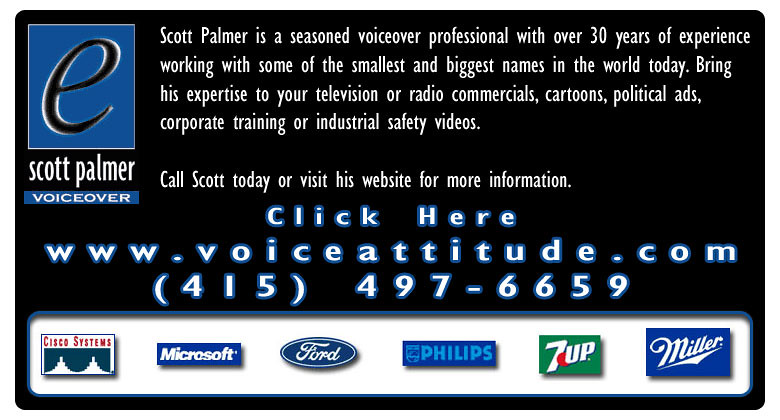This digital poster features a sleek black background with a prominent blue rectangle in the top left corner, housing a black cursive letter "E" bordered in white. Below this icon, the text "Scott Palmer" appears in white, followed by "Voiceover" in a thin blue rectangular box. To the right, a detailed white text reads, "Scott Palmer is a seasoned voiceover professional with over 30 years of experience working with some of the smallest and biggest names in the world today. Bring his expertise to your television or radio commercials, cartoons, political ads, corporate training, or industrial safety videos. Call Scott today or visit his website for more information." This is followed by a highlighted prompt in white with a blue outline that says, "Click here," directing viewers to "www.voiceattitude.com" and providing the contact number "415-497-6659." At the bottom of the poster, a white bar features the icons of renowned companies such as Cisco Systems, Microsoft, Ford, Philips, 7-Up, and Miller.